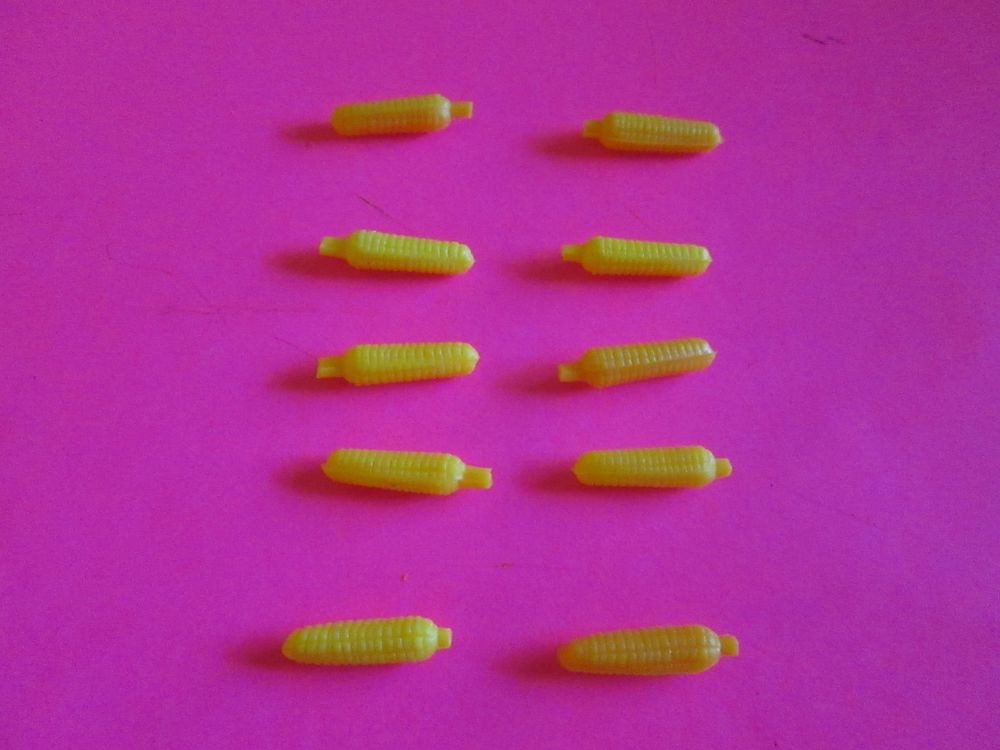This indoor photograph showcases 10 miniature plastic cobs of corn arranged on a smooth, bright magenta-pink background. Each cob, approximately an inch to an inch and a half in length and about a quarter inch in diameter, is injection molded from greenish-yellow plastic, displaying visible seams on the sides. The cobs are organized into two columns of five, spaced equally apart, with most of the husk portions oriented to the left and the pointed ends to the right. The corn cobs feature textured stripes that mimic individual kernels. The lighting, coming from the right, casts subtle shadows to the left. The image is in focus but slightly grainy, and no text or additional elements are present. These miniature cobs of corn could be part of a toy, model display, diorama, or dollhouse setup.